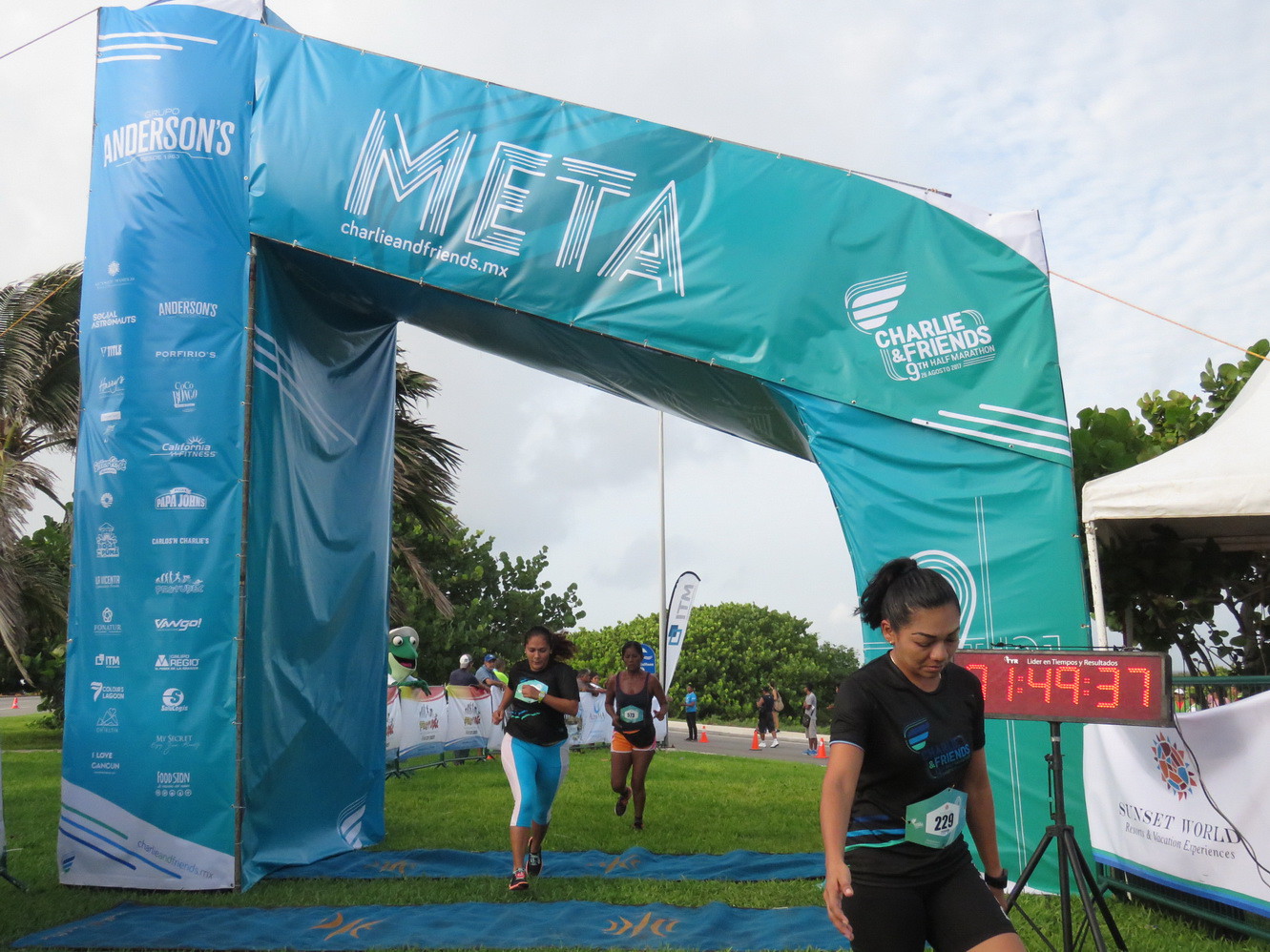The image captures an outdoor race, with runners crossing the finish line under a large, blue arch. The arch, made of tarp material, prominently displays the text "Meta Charlie and Friends.mx" at its top. In the foreground, a runner dressed in all black, with her dark hair tied up in a ponytail, is crossing the finish line to the right of a digital clock mounted on a tripod, which shows a time of 1:49:37. Blue tarps are laid out on the ground in front of the arch. Behind the arch, more runners approach the finish line, while spectators can be seen on the left side and in the background, where a road and grassy areas are visible along with some signs and poles. The sky is overcast, adding diffuse light to the scene.